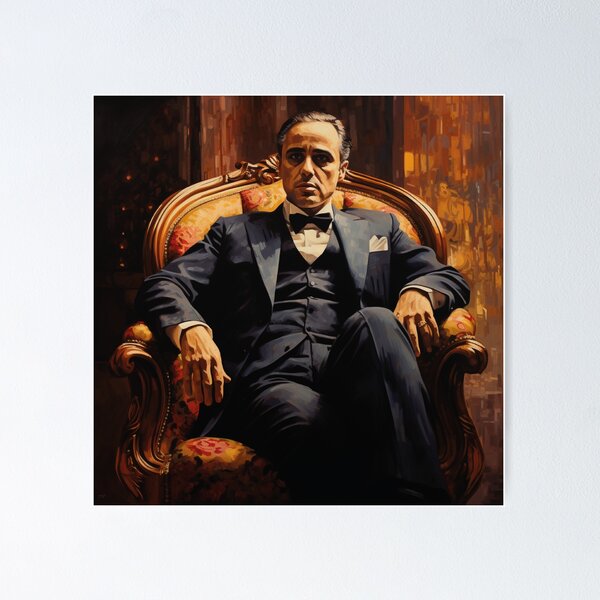The image depicts a textured light gray wall adorned with a square, oil painting print, thinly outlined in white with a subtle drop shadow. The painting showcases an iconic figure, unmistakably Marlon Brando's character, Vito Corleone, from The Godfather. Vito, an older, commanding Italian man with swept-back gray hair and a slightly shadowed expression, is seated in an ornate, high-backed chair with carved wooden armrests and a yellowish-red floral print cushion. He dons a sophisticated navy three-piece suit, complete with a navy vest, a white dress shirt, a black bow tie, and a white kerchief tucked into the breast pocket. The suit ensemble is paired with navy jeans, embodying the classic, powerful look associated with the character. The background behind him is a blend of bluish and brown hues, possibly depicting a draped window with light filtering through, adding to the atmospheric depth of the composition.